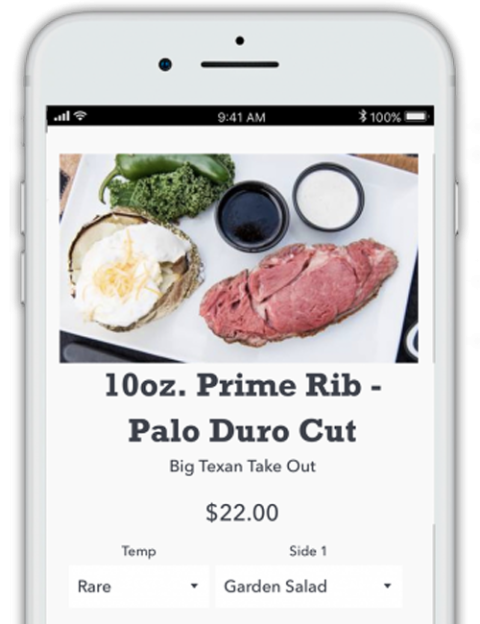A high-definition image displays a white smartphone showcasing a restaurant website. The top part of the phone screen features standard icons: signal strength, the time reading 9:41 AM, and a fully charged battery indicated by "100%." Below these, a vibrant photograph of a meal is prominently displayed, featuring an uncooked prime rib steak, a baked potato with skin, and what appears to be green vegetables such as possibly a jalapeño pepper, broccoli, and kale, all uncooked. The plate is accompanied by two small sauce dippers, one filled with a dark brownish-black sauce and the other with a white sauce.

Underneath the food image, text indicates the dish name: "10-ounce Prime Rib, Palo Duro Cut," followed by the label "Big Texan Takeout," all priced at $22. Further down, customization options are visible. The term "Temp" is followed by a drop-down menu currently set to "Rare." Next to it, a selection for "Side 1" is shown, defaulted to "Garden Salad," with an arrow signifying the presence of additional choices.